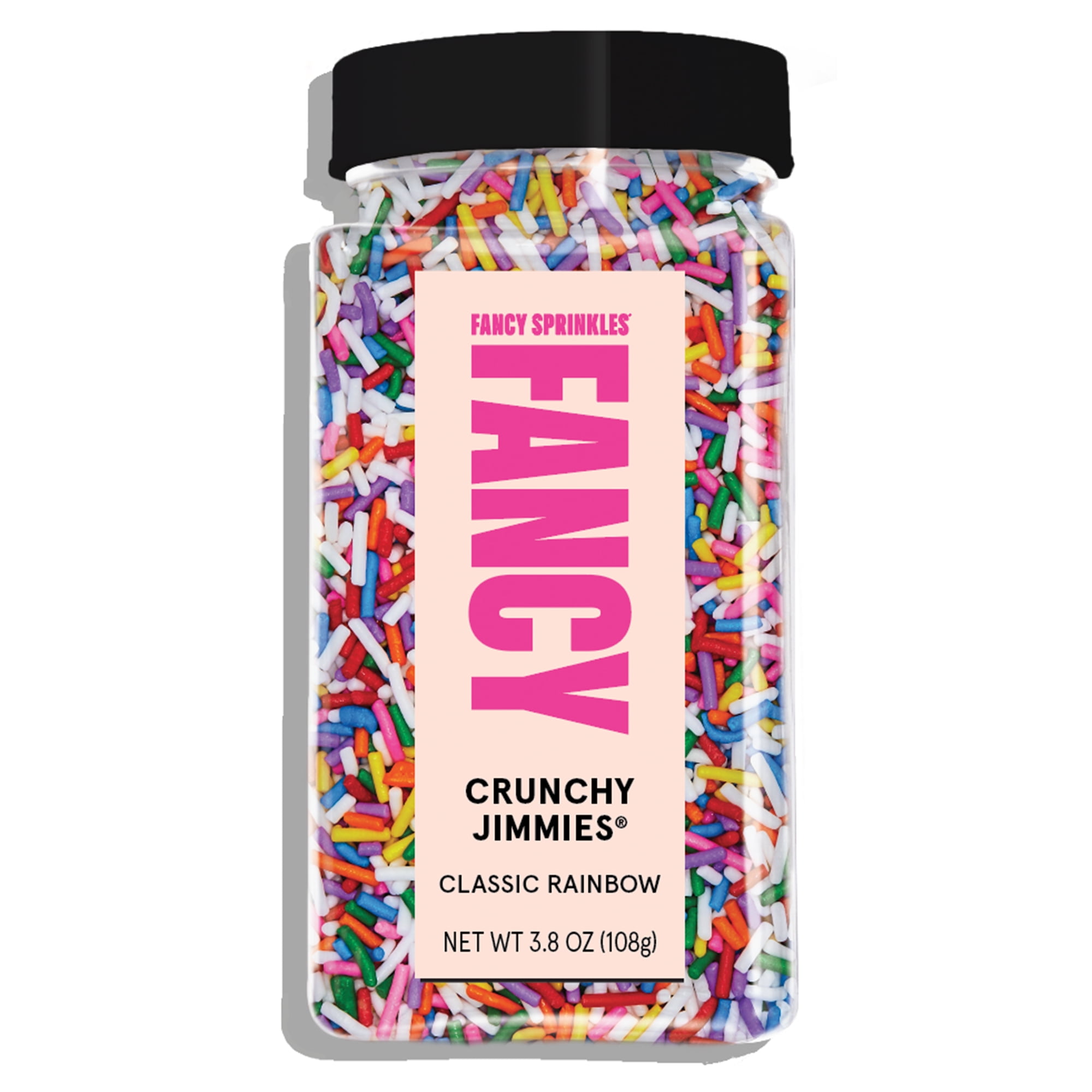The image shows a clear rectangular jar, either glass or plastic, with a black cap, containing a vibrant array of multicolored sprinkles. The label on the jar is light pink and reads "Fancy Sprinkles" in a small, dark pink font at the top. The word "FANCY" is prominently displayed vertically in large, magenta letters. Beneath it, in smaller black letters, the label reads "Crunchy Jimmies" and "Classic Rainbow." At the bottom, "Net Wt 3.8 oz (108 g)" is printed in black. Inside, the jar is filled with a colorful assortment of sprinkles in shades of yellow, pink, white, purple, red, green, blue, and orange, with numerous white sprinkles among the assortment.